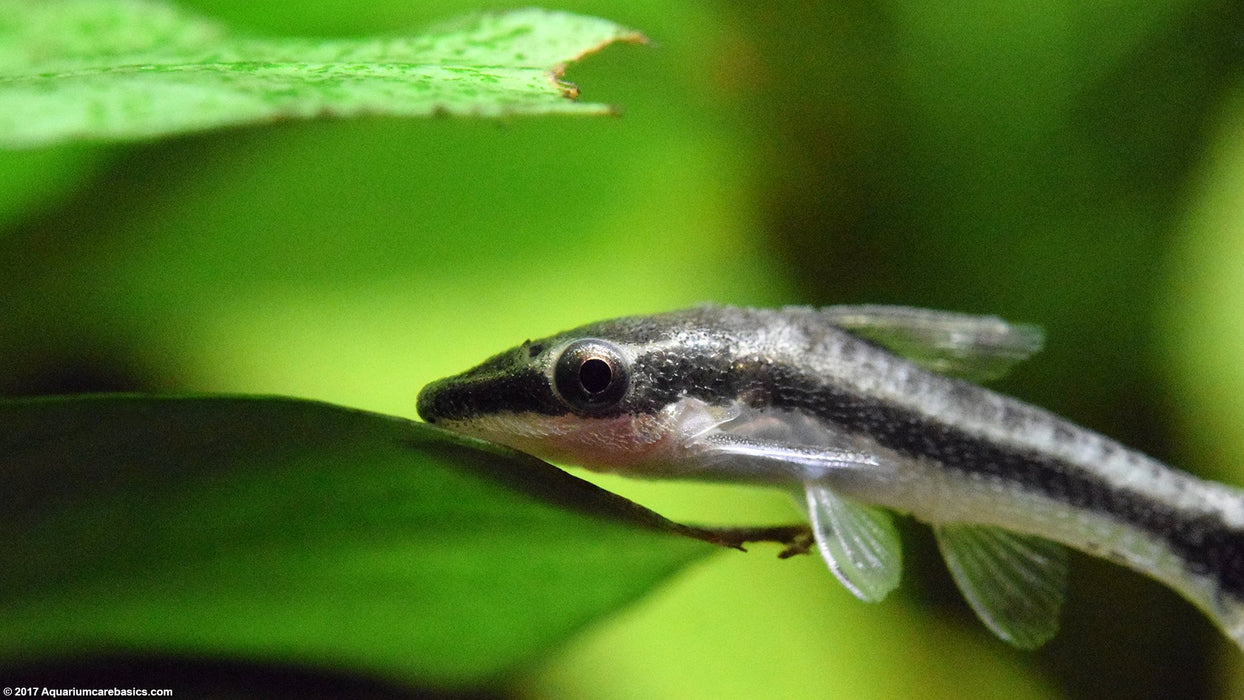This close-up photograph captures a small, thin, silver fish with a prominent, large eye staring directly at the camera. The fish showcases a distinctive black stripe running from its mouth to its tail, and its fins are nearly translucent. The underside of the fish displays a subtle pinkish hue near the mouth area. The backdrop is vividly green, resembling underwater vegetation, with various shades of leaf-green contributing to a lush, aquatic ambiance. The fish perches on or near leaves of a plant, adding to the tropical feel of the scene. In the bottom left corner of the image, the text "© 2017 AquariumCareBasics.com" suggests it might be an advertisement or an educational snippet about aquarium care.